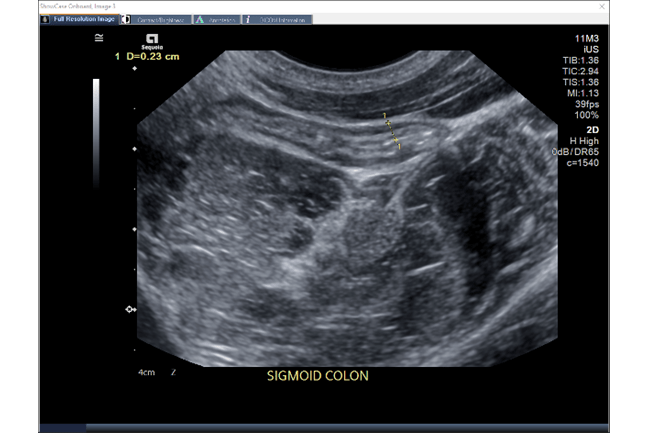The image depicts a black-and-white ultrasound with the curved top characteristic of sonographic images. Identified at the bottom, it is labeled as a "sigmoid colon," clearly revealing the anatomical focus. The ultrasound features a central vertical black area believed to represent parts of the colon, punctuated by a prominent white blob whose significance is indeterminate. The surrounding image is a mix of black with scattered white spots, typical of ultrasound scans. The on-screen display includes extensive text on the right, such as measurement annotations: "D = 0.23 centimeters" highlighted by a yellow line. Additional technical details are displayed: "11m3," "TIB 136," "TIC 294," "TIS 136," "MI 113," "39 FPS," indicating that the image was captured at 39 frames per second in high-resolution 2D mode at 100% scale. The ultrasound appears in a software interface with multiple tabs, suggesting a detailed and professional medical imaging setup.